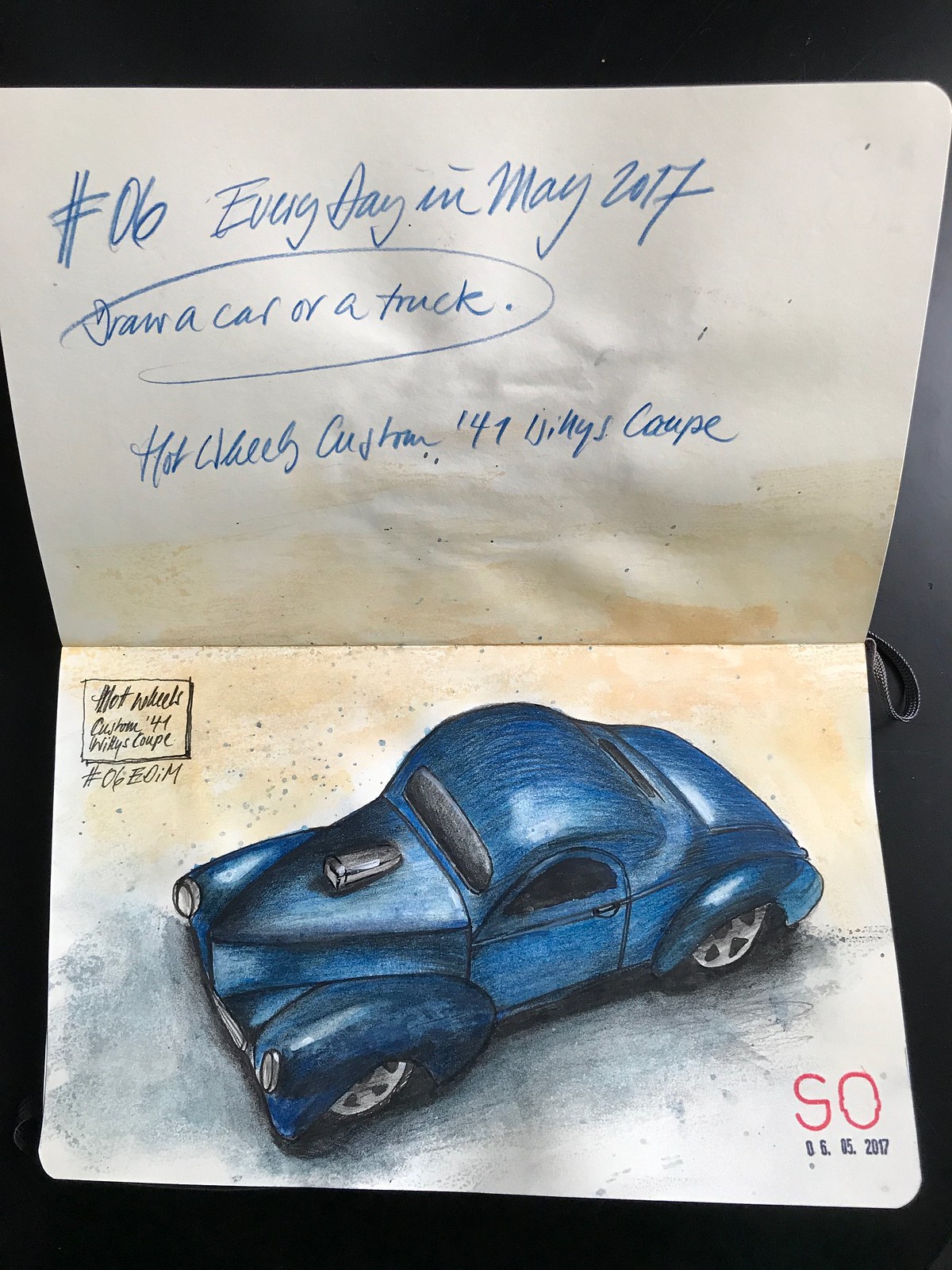The image showcases a picture of a blue retro-styled car, likely a Hot Wheels custom model, drawing inside a notebook that is opened to two pages. The car, possibly titled "Hot Wheels Custom 49 Wilkes Coupe number 606 EDIM" or a similarly named model, is small with distinct features: silver wheels, black-tinted windows, and triangular-shaped hood with silver headlights and front plate. The background around the car consists of blue and yellowish watercolor. The page above the drawing includes a handwritten note in blue ink that says "#06, every day in May 2017. Draw a car or a truck," with part of the text circled. The notebook is set on a black surface with light reflecting in the top right-hand corner.